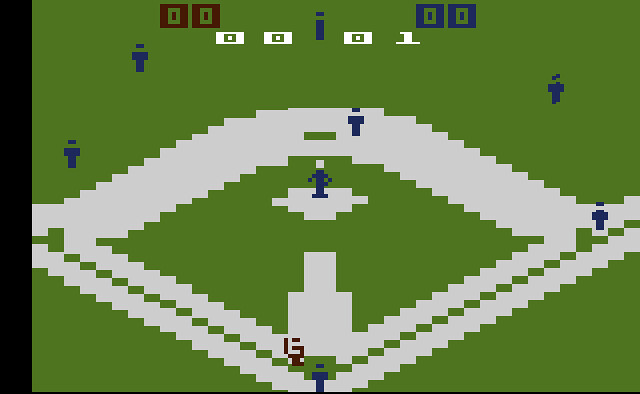This image is a nostalgic screenshot from a vintage baseball video game, likely from an era preceding iconic consoles such as Nintendo or Sega Genesis, suggesting it may be from systems like Atari or ColecoVision. The visual depicts a simplistic green field, with a basic white diamond representing the baseball diamond and a white mound at its center. The player at the plate is identifiable only by a red "G" logo. Meanwhile, the defensive players are rendered as blue stick figures adorned with blue numbers. Positioned prominently at the top of the screen, the game's score is displayed in red as 0-0. Beneath this, in white, are the numbers 0-0-0-1, with a blue character situated among them, featuring an eye-like shape for detail. This minimalistic yet evocative representation takes viewers back to the rudimentary yet charming days of early video gaming.